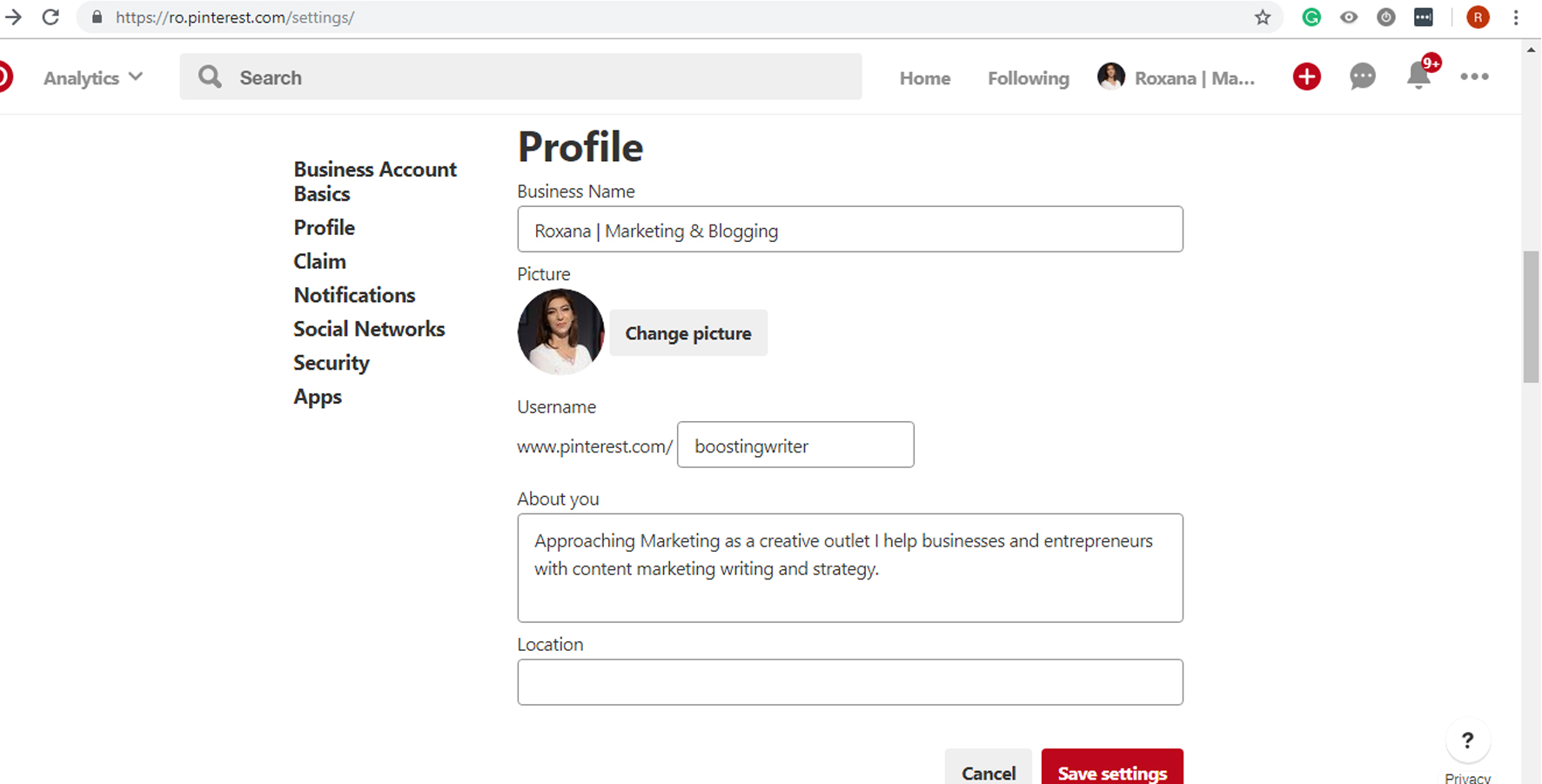The image is a horizontally rectangular screenshot of a Pinterest website displayed on a computer monitor. At the top of the screen, the web address "https://ro.pinterest.com/settings/" is visible. Directly below this, a menu bar displays options including "Analytics" with a dropdown button, a search field, "Home," "Following," and the individual's avatar. Next to the avatar, the name Roxanna is visible along with a notification icon indicating 9+ notifications.

The central focus of the screenshot is the "Profile" section, which is prominently displayed in the center of the screen. On the left sidebar, options such as "Business Account," "Basics," "Profile," "Claim," "Notifications," "Social Networks," "Security," and "Apps" are listed.

To the right of the sidebar, the "Profile" heading is bolded. Below this are various editable fields. The "Business Name" field is filled in with "Roxanna Marketing and Blogging." Beneath this is the option to "Change Picture," where the user’s current avatar is shown. The "Username" field displays "www.pinterest.com/boostingwriter." An "About You" section includes the following description: "Approaching marketing as a creative outlet. I help businesses and entrepreneurs with content, marketing, writing, and strategy."